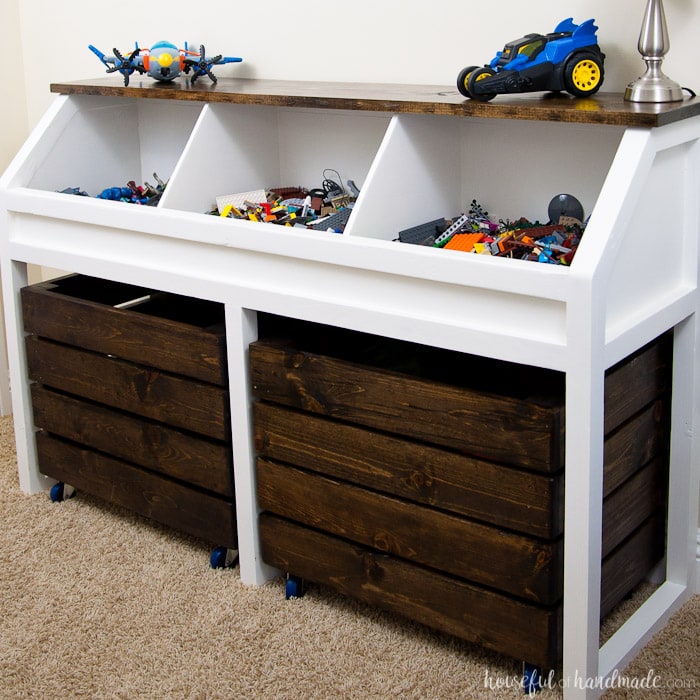This photograph from housefullofhandmade.com showcases an organized toy storage unit designed for children. The bottom section of the unit features two rustic wood crates on wheels, perfect for storing larger toys. Above these crates, the white desk-like furniture piece is divided into three open cubbies, meticulously categorized to hold various colorful toy pieces such as Legos, action figures, and building blocks. The shelves display completed Lego creations, including a vibrant airplane and a blue dune buggy with yellow interior wheels. The storage unit sits on tan carpet against light tan walls. The top shelf is adorned with a lamp placed next to the toy displays, adding a touch of practicality to the playful setup. The overall scene exemplifies an efficient and visually appealing method for organizing children's toys.